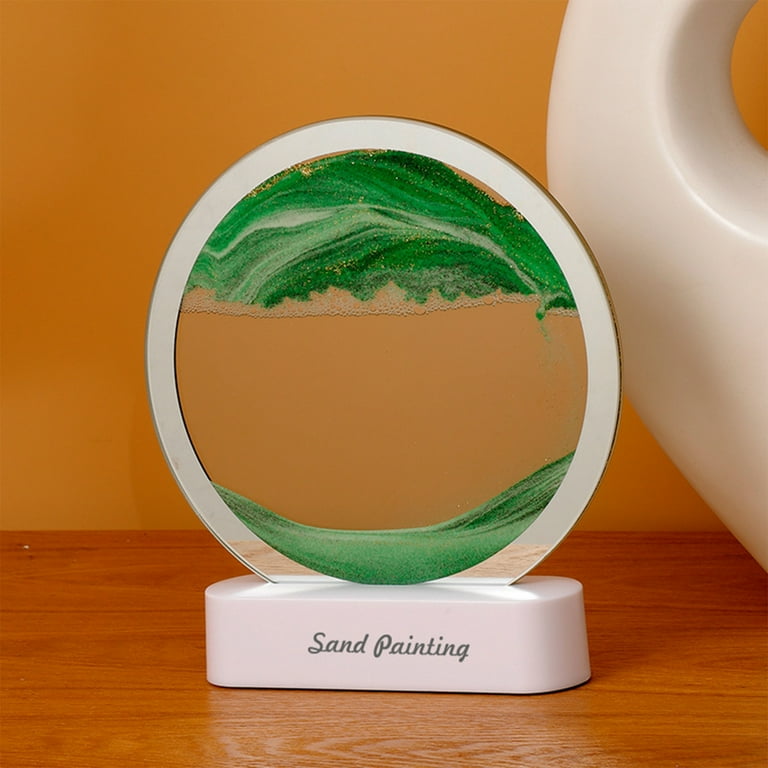The image features a decorative sand painting, prominently displayed on a wooden table against an orange, light brown, or caramel-colored wall. The painting is encased in a clear circular frame, which is supported by a pill-shaped base. The base has "sand painting" written in gray cursive writing. The circular frame appears metallic with a clear center filled with water and colored sand.

The sand painting is divided into two parts by a horizontal clear section that allows visibility through the glass. The upper part of the circle contains dark green sand, while the lower part holds a mixture of lighter green and tan-colored sand. Additionally, there are visible bubbles within this central clear section, suggesting the presence of water, which adds fluidity to the design and allows the sand to shift and create patterns. To the right of the sand painting, partially out of the frame, there is an indistinct white glass or ceramic object.